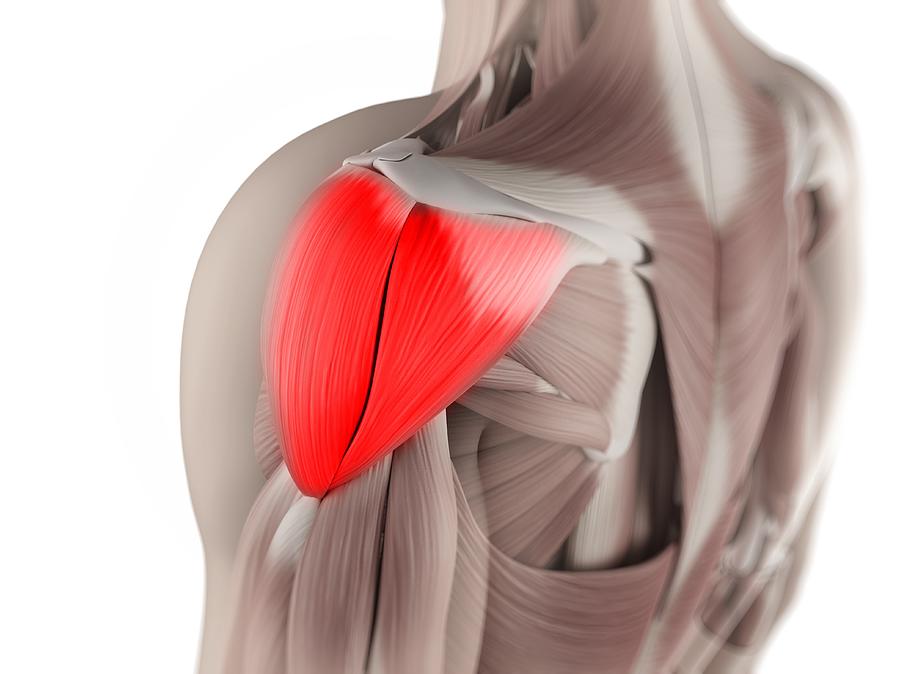This image presents a detailed 3D render of the human musculature, focusing primarily on the left shoulder. The rendering vividly showcases the deltoid muscle, prominently highlighted in bright red to suggest localized pain or significant anatomical importance. This muscle, appearing almost like a split tongue due to its natural division, is situated high on the shoulder and connects above by a joint or cartilage structure. The depiction transitions from the sharply defined shoulder muscles to the more blurred forms of the adjacent neck, back, and right shoulder muscles, creating a gradient of focus. The overall muscle coloration ranges from brownish-red to a bruise-like raspberry hue with areas of white, suggesting varying tissue densities and conditions. On the left, a narrow strip of skin delineates where the arm would extend, gently fading into the musculature. The background remains a stark white, accentuating the vibrant anatomical details.